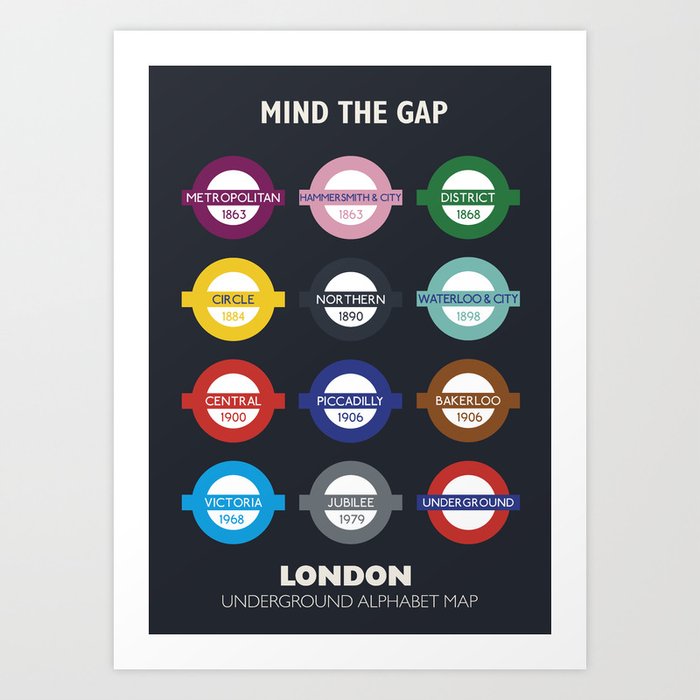This poster features a striking black background with a white border and trim, creating a bold frame for the central design. At the top, in crisp white lettering, it reads "Mind the Gap." At the bottom, also in white, it states "London Underground Alphabet Map." The core of the artwork showcases 12 colorful circles, each intersected by a horizontal line with the name of a London Underground line and the year it was developed in white text. Arranged in four rows and three columns, the circles include lines like the red 'Metropolitan' from 1863, the pink 'Hammersmith and City' from 1863, and the green 'District' from 1868. Additional lines such as Northern, Waterloo and City, Central, Piccadilly, Bakerloo, Victoria, Jubilee, and more follow, with each line distinguished by its unique color. The final circle features the iconic red circle with a blue horizontal line and white text that reads "Underground," symbolizing the entire network. This decorative piece is crafted in a style that makes it a likely find on art platforms such as Etsy.